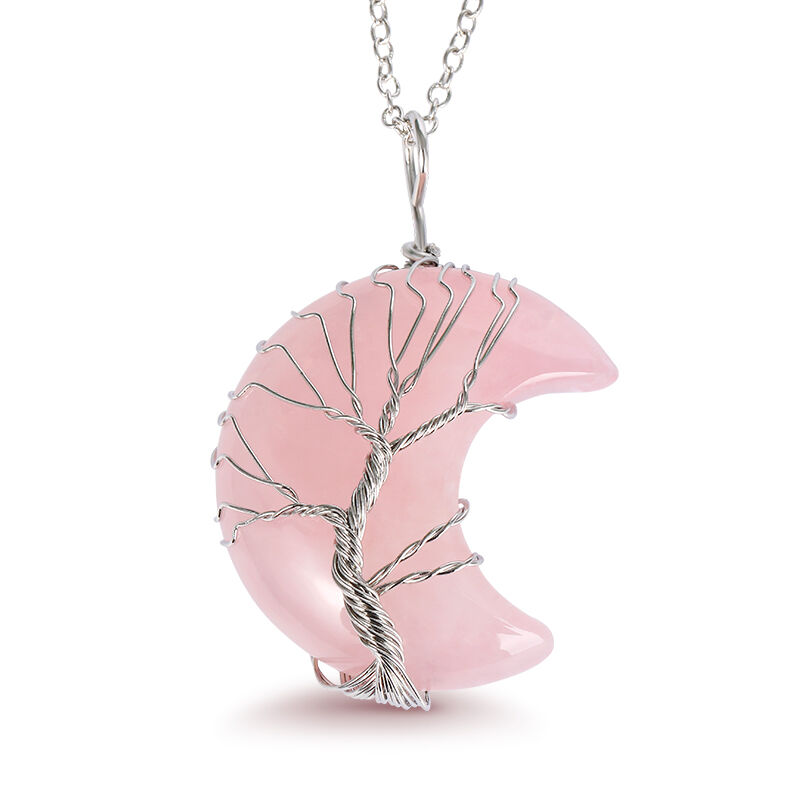This photograph showcases a delicate necklace set against an entirely white background. The necklace features a fine silver chain from which a pendant hangs. The pendant is intricately designed in the shape of a crescent moon, crafted from a light pink, shiny stone or gem, which could be glass or another material. The crescent moon is artistically wrapped with numerous strands of silver wire, approximately 20, creating the image of a tree. The main strand runs down the center serving as the trunk, while the other strands branch out, surrounding the moon-shaped pendant. The silver chain is connected to the pendant by a silver loop, and light reflects off the pink moon piece, highlighting its luster.